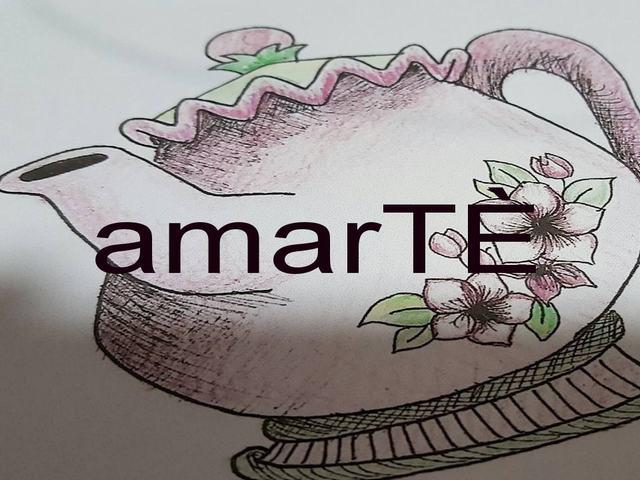The image is a detailed, illustrated drawing of a white teapot with a pink handle and decorative elements, set against a white background that resembles a piece of paper. The teapot features a lid with a circular knob on top, adorned with green grass-like or petal designs. The body of the teapot displays two partially bloomed flowers with green leaves and unbloomed buds. Black shadowing and cross-hatching provide depth and texture, particularly evident at the bottom and around the handle. The text "Amarte" is inscribed on the teapot, with the letters styled in lowercase for "amar" and uppercase "TE" with an accent on the "E". The teapot's spout and sections near the base are shaded, incorporating pink and black bordering around the flowers, with checkerboard and vertical line patterns enhancing the design at the bottom. The teapot is slightly slanted to the left within the image frame, which has a simplistic, clean background.